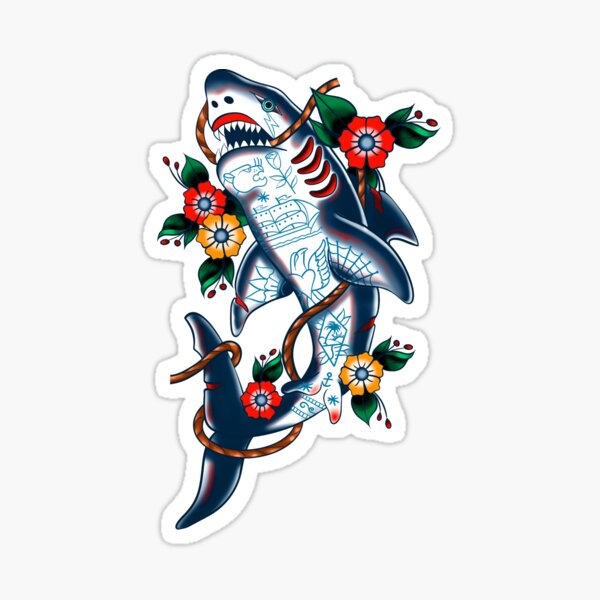This image portrays a large, vividly colored shark with a dynamic, swirling posture suggestive of motion. The shark has a blue and white body, with its mouth open, revealing sharp teeth and red gums. Green eyes and a caramel-colored rope wrapped around its mouth and lower body add to its detailed design. The shark’s body is adorned with various blue stick drawings, including musical notes, a lion, a bird, a heart with wings, and puma-like figures. Its fins feature intricate elements such as spider webs and arrows.

Surrounding the shark are several vibrantly colored flowers: two red flowers at the top, accompanied by a yellow or orange flower beneath the left one, a yellow flower at the bottom right, and another red flower near the tail on the bottom left. Each flower is detailed with green leaves.

The entire image appears to be encased in a thick white outline, giving it a distinctive sticker-like appearance. This could be seen as a design suitable for a tattoo, a skateboard sticker, or an eye-catching label. The overall impression is of a brightly colored, cartoonish shark surrounded by flowers, perhaps whimsically attempting to brighten someone's day despite its formidable appearance.